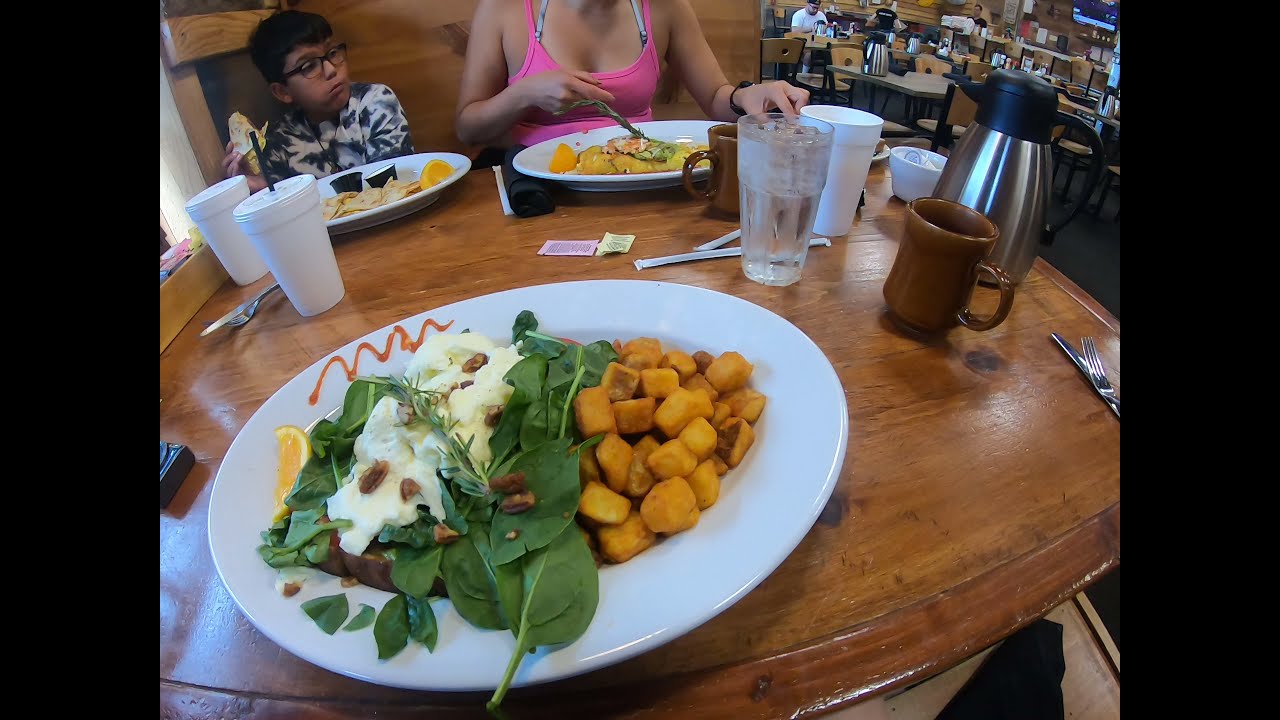This photograph captures a bustling restaurant scene from the vantage point of someone seated at a booth, which features a medium brown, glossy wooden table. The table, curiously curved due to a special lens, dominates the foreground. At the far end, a child and a woman are seated. The child, with light brown skin, short black hair, and black glasses, sports a blue tie-dye shirt and is focused on a white tortilla-like food on his oval-shaped white porcelain plate. To his right is a woman with light brown skin, donned in a pink thin-strap tank top with a bikini top or gray bra underneath. The table is scattered with dining essentials, including round white porcelain plates, which feature a variety of foods such as fried potatoes, lettuce, mashed potatoes on toast, chopped carrots, and a brown sauce dribbled decoratively. In addition, there are white Styrofoam cups, brown coffee mugs, a clear glass of ice water, a silver coffee carafe with a black top, silverware, straws, and artificial sweetener packets. The restaurant’s environment is partially visible, showcasing other brown tables, various patrons, and a television set in the upper right corner. The image itself is cropped with black vertical bars on both the left and right sides.